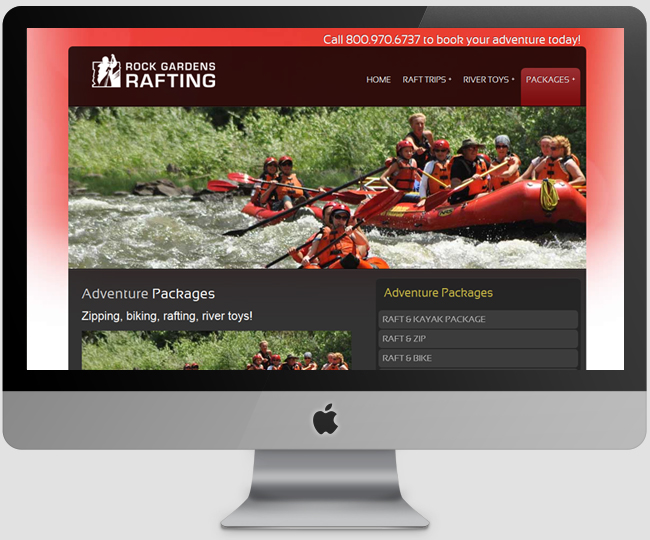A vibrant advertisement or website for "Rock Gardens Rafting" is showcased against a mostly white background. In the top left corner, bold text reading "Rock Gardens Rafting" is accompanied by enticing images of white water rafting and lush green grass. Below it, an invitation to "Call 800.970.6737 to book your adventure today" is prominently displayed. This section also includes a series of tabs titled "Home," "Raft Trips," "River Toys," and "Packages," illustrated with respective icons.

In the center, an engaging scene unfolds: a group of adventurers paddling through thrilling rapids in white water rafts, adorned with colorful safety vests and fins. Further to the right, more people can be seen inside their rafts, battling the rushing waters.

The bottom left corner features additional enticing options with labels such as "Adventure Packages," "Zipping," "Biking," "Rafting," and "River Toys," all presented over a backdrop of verdant green grass. 

The borders of the advertisement highlight different package deals: "Raft and Kayak Package," "Raft and Zip," and "Raft and Bike." An image of an iMac rests on a silver stand in the back border, with recognizable icons of a red apple and silver details at the bottom, hinting at a seamless digital booking experience.

Overall, this compelling layout captures the essence of exhilarating river adventures, urging thrill-seekers to plan their next escapade with Rock Gardens Rafting.